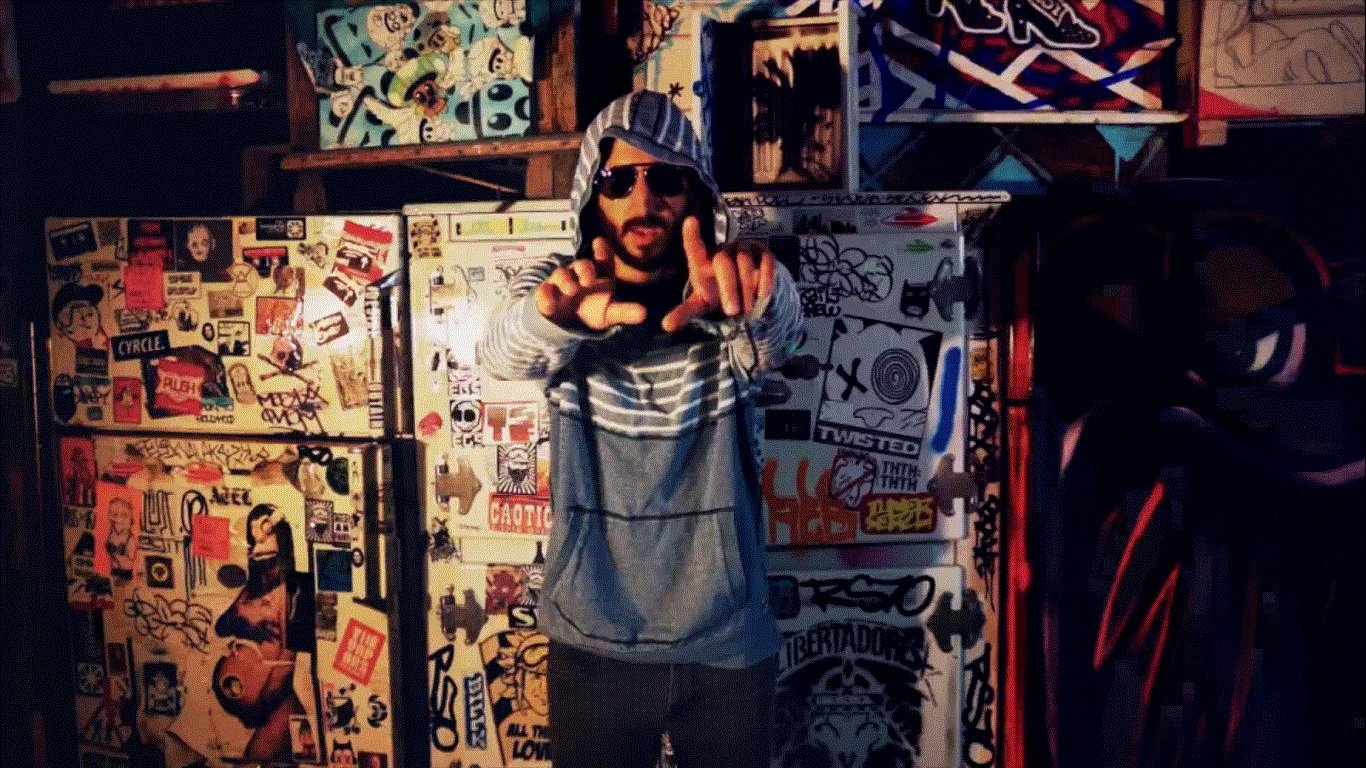In a dimly lit, basement-like area, a man stands central in a color photograph, facing the camera. Behind him, three white refrigerators, extensively covered with an eclectic mix of stickers, magnets, and possibly graffiti, dominate the background. There's scarcely any white surface left visible on the fridges. Above them, wooden shelves with more stickers or graffiti add to the cluttered and urban ambiance. The man, exuding a hipster vibe, wears dark-colored jeans and a gray hooded sweatshirt. The top portion of the sweatshirt, including the chest, sleeves, and hood, is adorned with white stripes. He completes his distinct look with a dark beard, mustache, and dark aviator-style glasses. His hands are held out towards the camera with both pointer fingers extended and nearly touching, forming an "L" shape. The image captures a moment that feels steeped in pop culture and nostalgia.